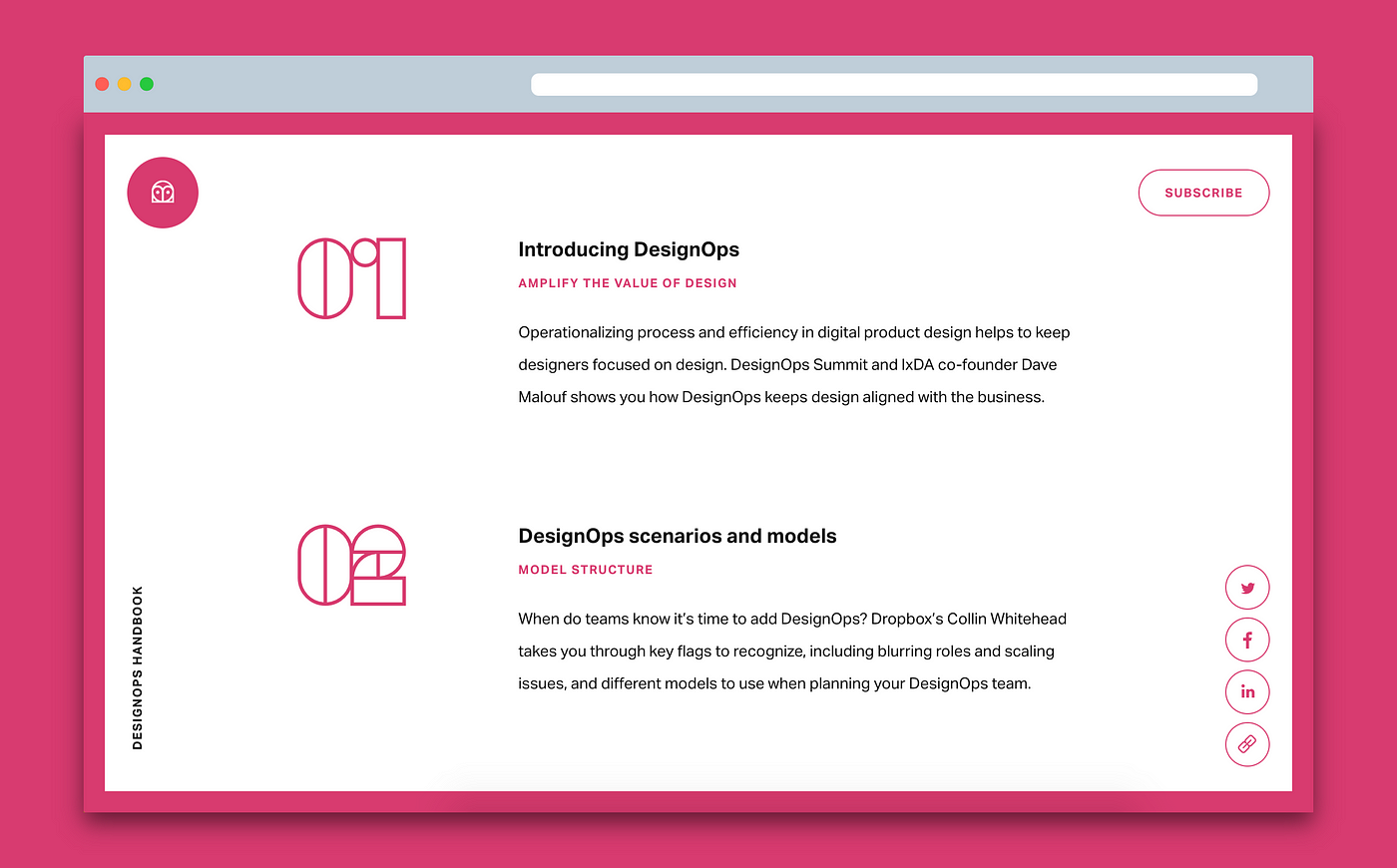This detailed caption describes a horizontal screenshot featuring a vibrant pink border around the entire image. The screenshot is dominated by a gray header bar at the top, which includes three colored dots (red, yellow, and green) on the upper left-hand corner, typical of a web browser or application window. Noticeably, there is no address bar, and instead, there is an elongated white space in that area.

Within the main section of the image, at the upper left-hand corner, there is an icon enclosed in a pink circle. The center background is stark white, providing contrast for the content. Prominently displayed in an elegant typeset are two large numbers, "01" and "02," each followed by respective headings. 

The first heading, "Introducing Design Ops," includes bright pink subtext that reads, "Amplify the Value of Design," with an accompanying paragraph beneath it. The second heading, "Design Ops Scenarios and Models," features subtext in pink that states, "Model Structure," followed by another paragraph.

In the upper right-hand corner of this white section is a subscribe button. Along the lower left-hand side, written vertically and moving from the bottom up, the text "Design Ops Handbook" is displayed. 

At the lower right-hand corner, there are icons for Twitter, Facebook, Instagram, and a generic link, indicating options for sharing or further exploration on social media platforms.